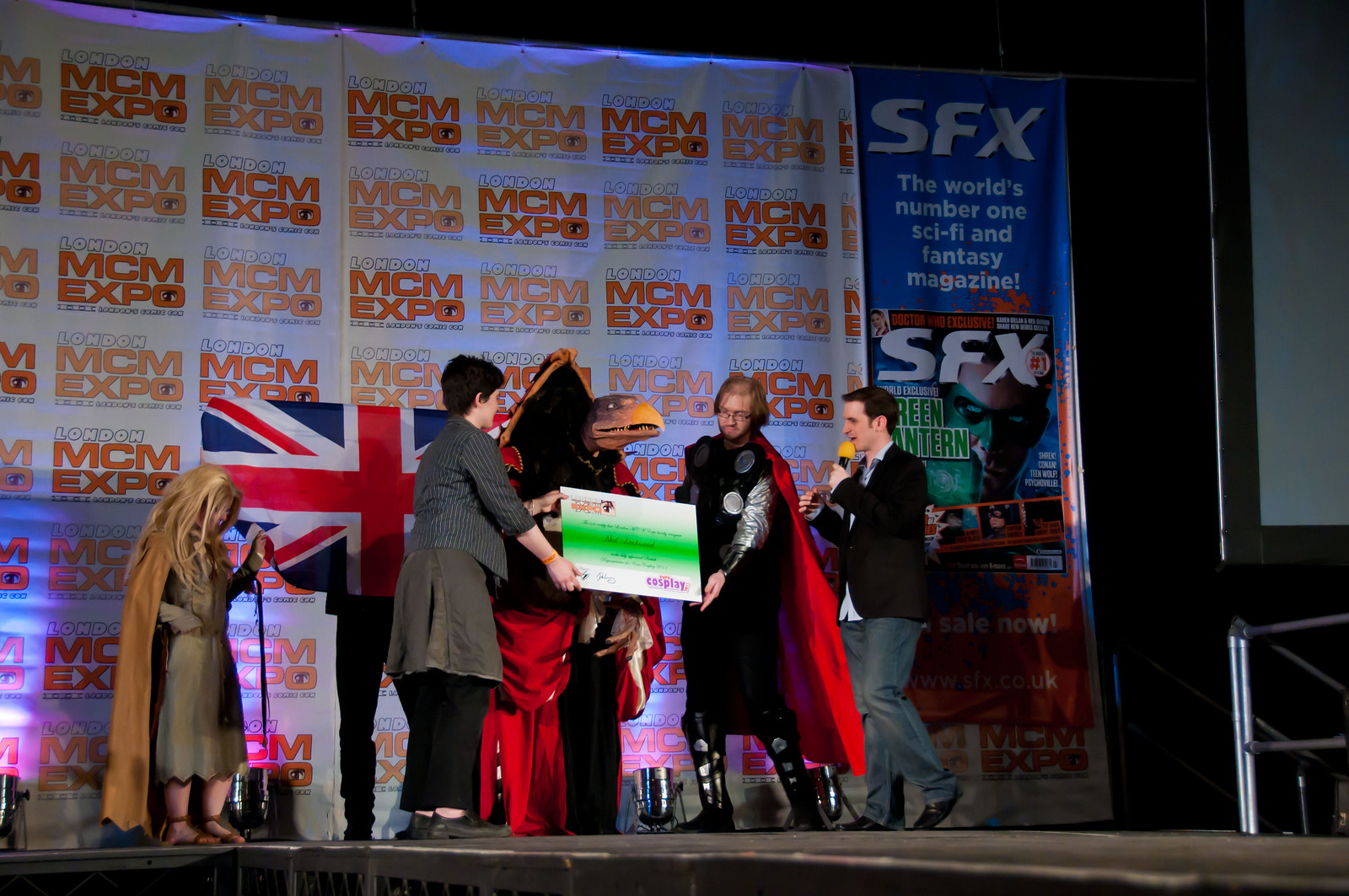This photograph captures a dynamic scene on a stage at the London MCM Expo, where an award presentation is taking place. The stage is bustling with four individuals, each dressed in elaborate costumes. Central to the image is a person in an intricate bird costume from Jim Henson's Dark Crystal, flanked by two others. One of them is a man dressed as Thor, wearing a black outfit, a red cape, and black and silver boots, while the other figure in a red cape holds the award alongside Thor. The award features a green bar gradient and bears the MCM Expo logo, along with the word "Cosplay" in purple.

To the left of the stage, a woman with long blonde hair, clad in a brown dress and cape, stands at a microphone. She appears to be announcing or facilitating the presentation. Behind them, the backdrop is a white banner adorned with the repeating text "London MCM Expo" in red and green, with a British flag adding to the scene's atmosphere. The lower part of the stage floor is visible, displaying an older, dark gray surface, while a large screen looms in the upper right corner, though it remains unlit. The overall image reflects the vibrant and celebratory nature of this cosplay award event.